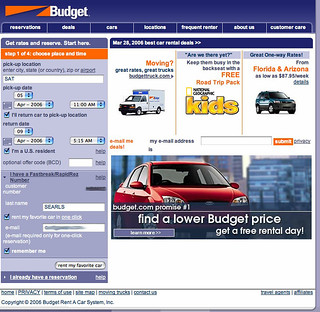Screenshot of Budget Rent-A-Car Website

The image is a square screenshot of the Budget Rent-A-Car website, likely taken on a computer or laptop rather than a mobile device. The background features a thin lavender border along the right side and bottom edges. Dominating the screen is the web page itself.

At the top of the page, there's a thick blue banner with the Budget logo prominently displayed on the upper left-hand corner in orange and white. Situated within the banner are several navigational tabs, including Reservations, Deals, Cars, Locations, Frequent Renter, About Us, and Customer Care.

Central to the page are booking details titled "Get Rates & Reserve," marked as Step 1 of 4: Choose Price and Time. The blurry text suggests that the user—a U.S. resident—intended to pick up a car on April 5, 2006, at 11 a.m. and return it on April 9, 2006. Despite the blurriness making it difficult to confirm the exact dates, the information conveys the user's booking timeline.

Additionally, the image includes an advertisement, featuring a red sedan and a moving truck, showcasing Budget's vehicle offerings.